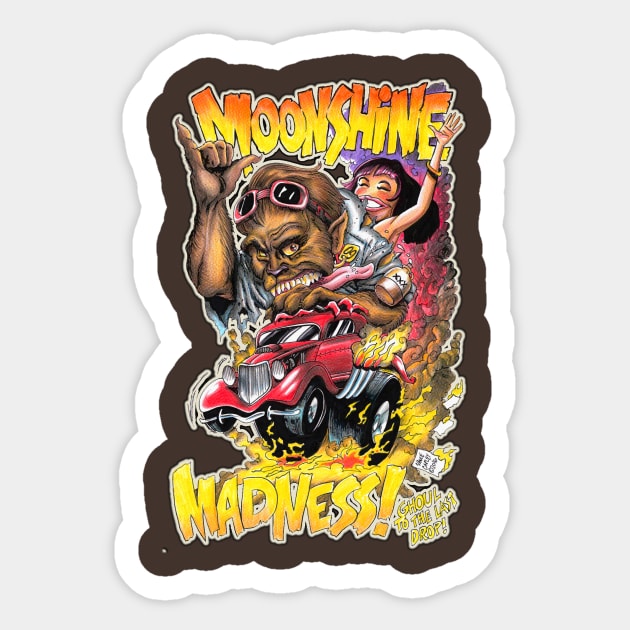This vibrant and wild poster titled "Moonshine Madness" features an electrifying and chaotic scene. Dominating the composition is a monstrous, werewolf-like creature with brown skin and sharp upper teeth, driving a compact dragster that appears almost too small for its hulking frame. The werewolf, whose long tongue dangles out and whose eyes are hidden by pink-rimmed goggles perched on its forehead, exudes a menacing yet cartoonish aura. Its right arm is raised, hand positioned with the center three fingers down and the thumb and pinky out, while its other clawed hand fiercely clutches the dragster's wheel. Flames and smoke billow dramatically from the rear of the vehicle, adding to the fiery intensity of the scene. 

Behind this fearsome driver stands a woman with light beige skin and black hair that has a hint of purple at the front. Her hand is outstretched, and a sly smile graces her face, contributing to the poster's chaotic energy. A traditional moonshine jug marked with three X's is also present, reinforcing the theme. 

At the top of the poster, the word "Moonshine" is prominently displayed in large, yellow text with an orange outline, while at the bottom, the word "Madness" follows in similarly bold yellow letters with an exclamation point. The tagline "Go, G-H-O-U-L to the last drop" adds a creepy-cool touch. Encasing the entire scene is a brown border followed by a white one, set against a very light gray background that makes the colors pop. This brilliantly detailed artwork captures the wild and frenetic spirit of "Moonshine Madness."